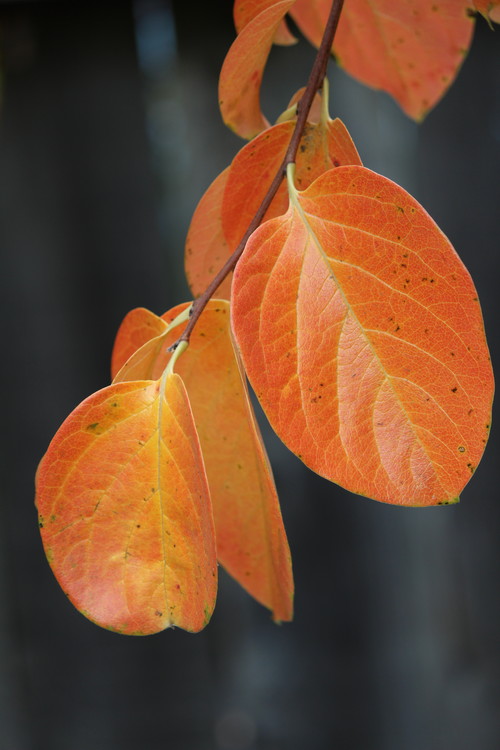This close-up photograph captures an autumnal scene of a tree branch with elongated, heart-shaped leaves. The main subject, a dark chestnut brown twig, protrudes downward into the frame against a blurred bluish-gray and black background, giving the image a soft, out-of-focus backdrop. The reddish-brown twig supports approximately 6-8 significant leaves, which are bright orange with some brown speckles, reminiscent of the color of an apple. Each leaf showcases a central vein, with lighter yellow and green lines branching off. Prominently, a large leaf dominates the right side of the image, while another sizeable leaf hangs at the very tip of the stem, accompanied by two more nearby. Additional leaves extend towards the top of the picture, contributing to the vibrant autumnal display.